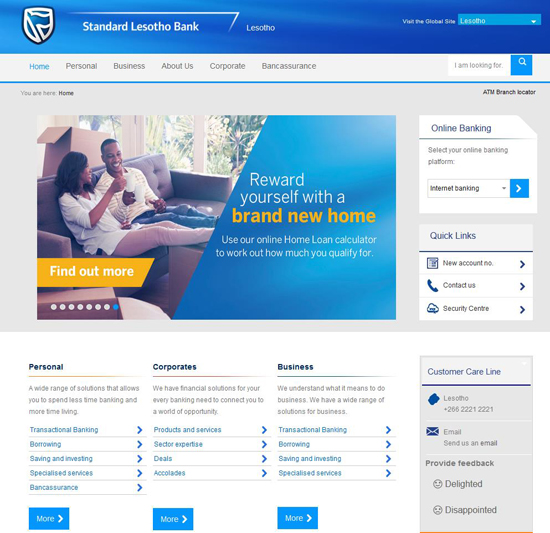This screenshot features part of the website for Standard Lesotho Bank, Lesotho. The top of the page displays a blue banner adorned with a grey crest logo on the left side. Next to the logo, in white text, are the words "Standard Lesotho Bank, Lesotho." On the upper right-hand corner of this banner is a blue search bar.

Beneath the blue banner, the primary background color of the page is white, accented by a blue horizontal line. On the left side of this section, there are several tabs. The "Home" tab is highlighted in blue, indicating it is currently selected. Next to it in grey text are additional tabs labeled "Personal," "Business," "About Us," "Corporate," and "Bancassurance."

Further down the page, there is another search box with a blue search button to the right. Below this, an image captures a relaxed scene: a man and woman of dark skin tone sitting on a couch. Both are clad in light-colored tops, the woman wears beige trousers while the man sports blue jeans and a long-sleeve lined shirt. The woman appears to be holding something up in her hand. Behind them, there is some greenery visible through a window to the upper right, and a cardboard box sits on the couch behind them. Within the image, there’s a yellow rectangle at the bottom with white text stating, "Find out more."

To the right of the image, a blue background presents white text, "Reward yourself with a brand new home," with "a brand new home" highlighted in yellow. Below this, a prompt advises using the online home loan calculator to determine loan qualifications.

The right side also features several essential links including "Online Banking," "Quick Clicks," "New Account Number," "Contact Us," and "Security Centre." Below these links are tabs for "Personal" and "Corporate Business," suggesting various banking services. The lower right-hand corner displays customer care line numbers for additional support.